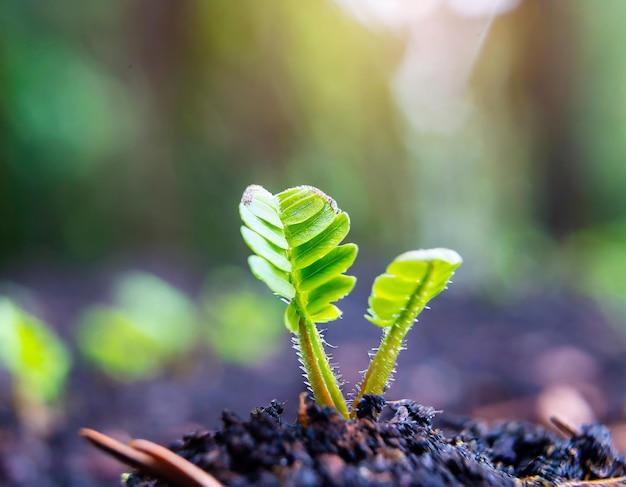In this vibrant landscape photograph, the focal point is a young sprout delicately emerging from a small mound of rich, brown soil. The sprout, adorned with tiny green leaves and fine white hairs along its stems, stands prominently in the sharp, detailed foreground. The soil also features twigs and little bits of corn. Surrounding the sprout are green branches with leaves, hinting at other seedlings preparing to emerge. In the blurred background, a forest scene unfolds, with indistinct trees and patches of greenery, all bathed in soft streams of sunlight filtering through the foliage. The overall image captures a vivid interplay of colors and textures, from the earthy brown ground to the lush green of the new growth, highlighting the tender resilience of life sprouting amidst the forest.